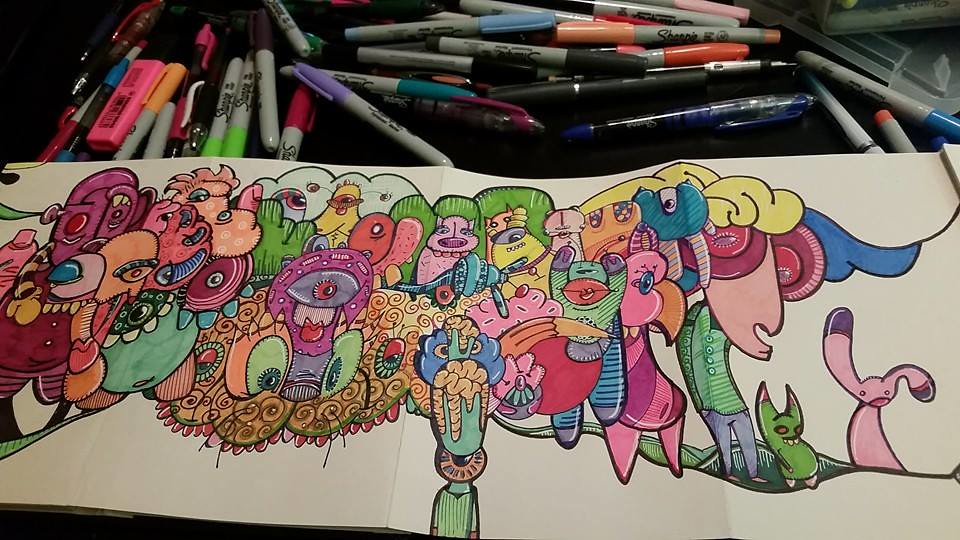The image features a wide, horizontally-oriented piece of paper adorned with vibrant, multicolored artwork. The artwork comprises an eclectic array of unusually designed creatures, depicted in a rich palette that includes yellows, blues, pinks, greens, purples, and other colors of the rainbow. Among the whimsical characters, there is one with a large head adorned with wide hair and big eyes, yet possessing a human body. Another distinctive figure is a pink bunny that lacks arms and has floppy ears. These quirky, animal-like designs, varying in appearance and color, populate the foreground, each exuding a unique charm.

Above this colorful scene, a black tabletop is visible, scattered with Sharpie permanent markers in an assortment of shades such as purple, pink, blue, orange, black, and green. The presence of these markers hints at the medium used to create the imaginative artwork below.